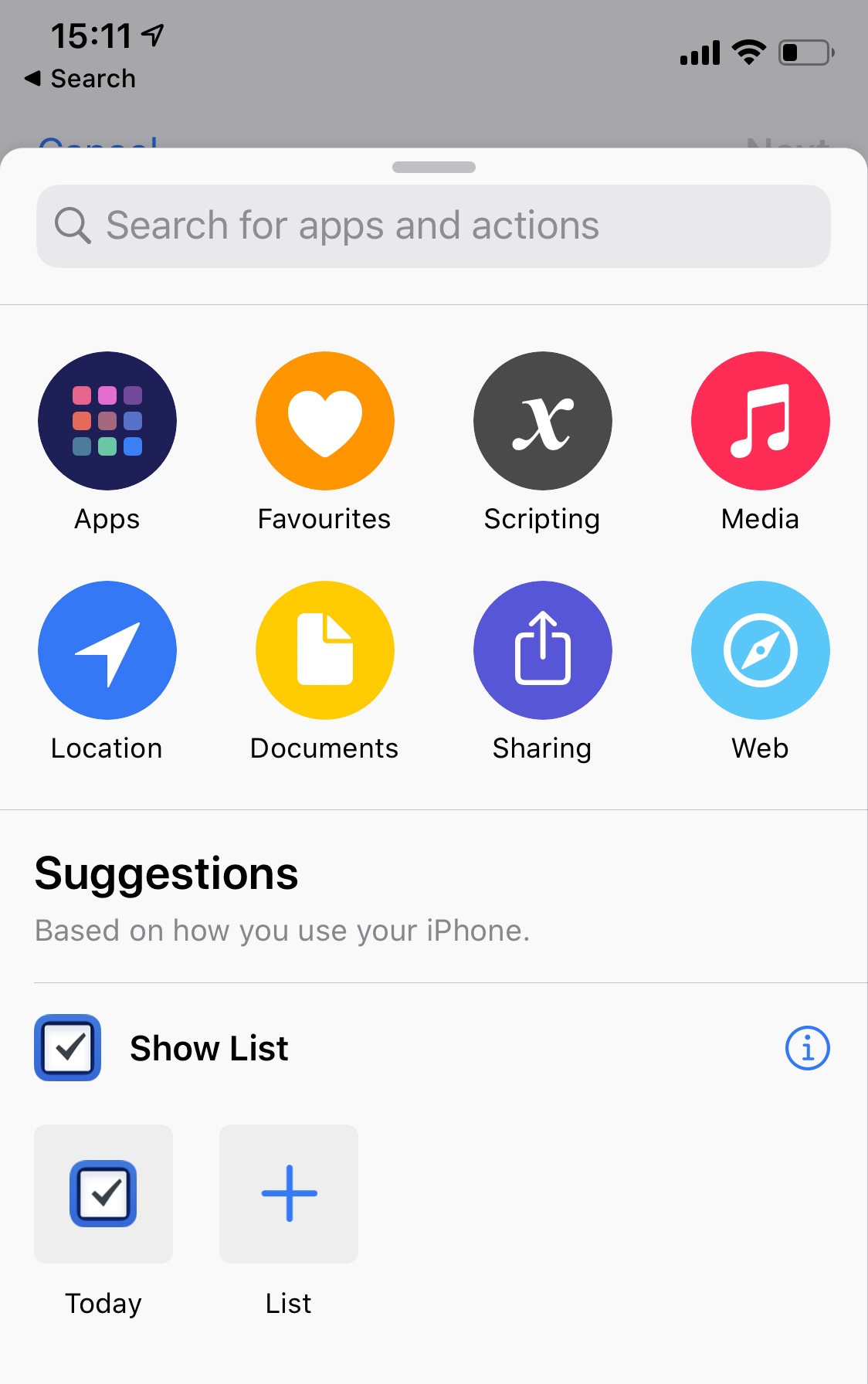The image depicts a snapshot taken from a cell phone screen, likely showcasing a feature or app interface. At the top of the screen, the status bar displays a gray banner with black text. On the left side, the time is indicated as 15:11. Adjacent to it is a diagonal upward-facing arrow. On the right side of the banner, icons for cell signal, Wi-Fi, and battery status are visible.

Beneath the status bar, there is a back arrow icon pointing to the left, labeled "Search" with a capital 'S'. Some blue text is partially visible at the bottom, though it is cut off by what appears to be a pop-up overlay.

The pop-up overlay is white with a thin gray line at the center top, indicating it can be dragged. Below this, there is a lighter gray search bar containing a magnifying glass icon and the text "Search for apps and actions".

The interface features two rows of circular icons. The first row contains four icons labeled as: 
- "Apps"
- "Favorites"
- "Scripting"
- "Media"

The second row also has four icons labeled as:
- "Location"
- "Documents"
- "Sharing"
- "Web"

Further down, bold black text reads "Suggestions," followed by the description "based on how you use your iPhone." Below this, there are more interface elements: a square with a black checkmark labeled "Show List," and a blue circular icon with a lowercase 'i' inside, indicating info.

On the left side of the screen, there are two labels: "Today," which is marked with a blue square containing a black checkmark, and "List," marked with a blue plus sign. These likely represent different categories or sections within the app.